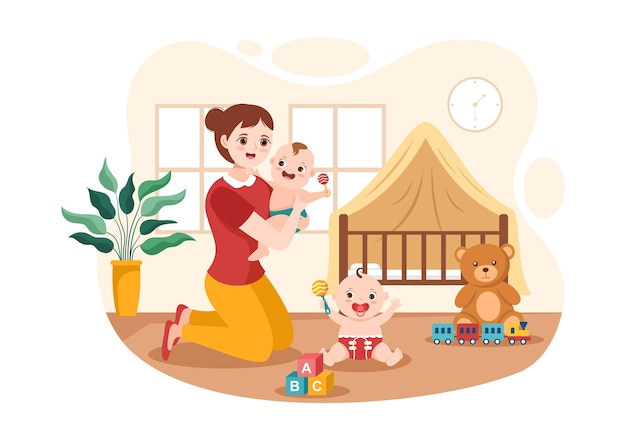In a cozy nursery, a young mother dressed in a red top, yellow pants, and red shoes with a white collar and her brown hair pulled back in a bun, is holding one of her twins. The baby, in a green diaper with a single slick curl on his head, clutches a baby rattle. Despite her tired eyes, the mother's smile radiates joy as she spends time with her children. The other baby, in a red diaper and also with a single slick curl, sits on the floor happily playing with a yellow rattle and using a red pacifier. The nursery's warm atmosphere is enhanced by a wooden brown crib draped with a tan canopy, a large teddy bear, and a colorful toy train at the crib's foot. Scattered on the brown floor are ABC building blocks in red, blue, and yellow. On the wall, a clock reads 2:30 in the afternoon, suggesting nap time is near. The room also features two simple windows and a modest green potted plant with a yellow base. The digitally created cartoon-style drawing captures the tender interaction between the mother and her twin babies, framed by the inviting and playful setting of their nursery.